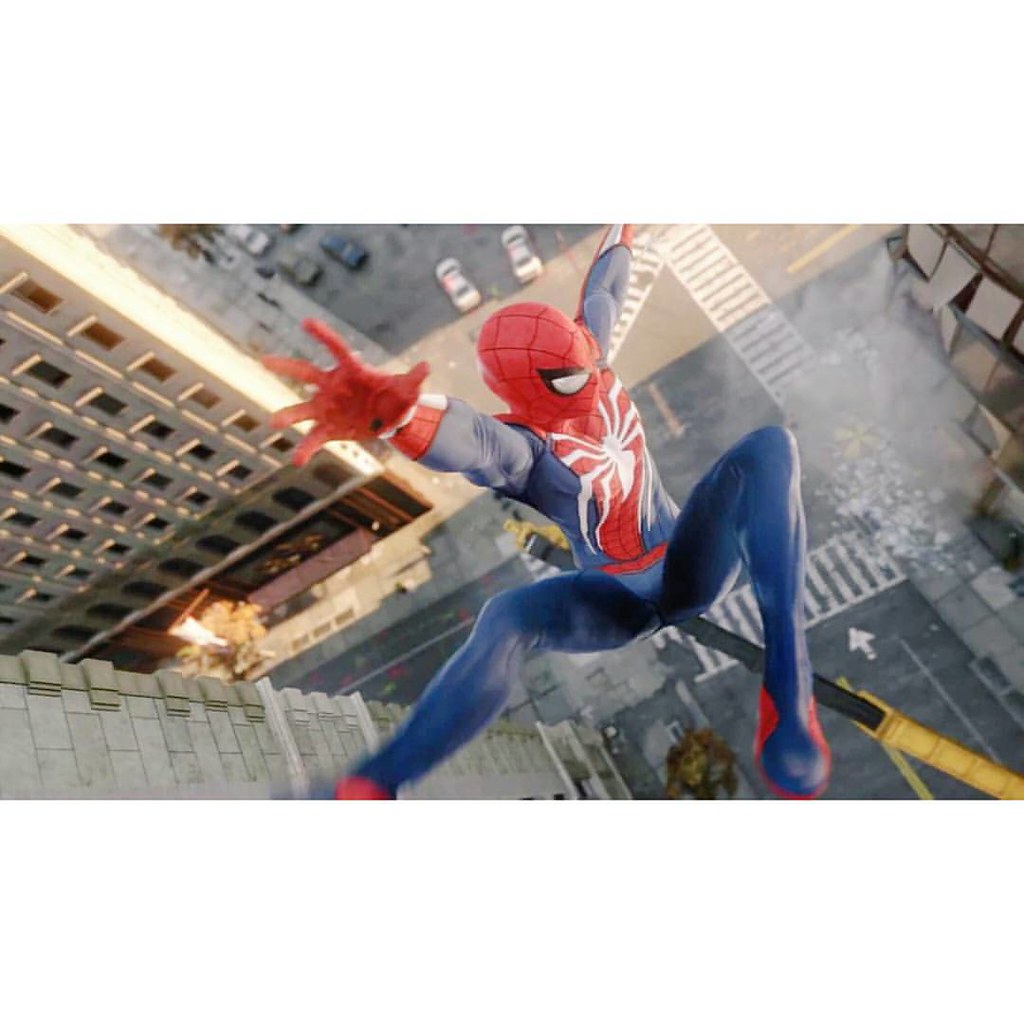This image is a detailed and dynamic screenshot from a Spider-Man video game, showcasing Spider-Man suspended approximately 20 stories high above a bustling street scene. The perspective is from above Spider-Man, who is captured mid-action with his arms and legs spread out. He appears to be either flying between the buildings or in the process of falling. Spider-Man is dressed in his classic red and blue suit with a white spider emblem on his chest and is wearing his iconic Spider-Man mask and red gloves.

In the intricate backdrop, several buildings are visible, including one resembling an office building and another that looks more like a federal building. To the right-hand side, there's a notable accident scene where the facade of a building has been partially blown off and debris is scattered on the street below. A yellow crane stands prominently in the background, adding to the urban complexity. Several cars, including two white ones, can be seen on the road, along with a few trees adding greenery to the cityscape. Additionally, a white directional arrow is visible on the street below Spider-Man. To the upper left, there is a parking lot with more cars, and some of the surrounding buildings have dark windows, suggesting unoccupied or internal spaces. The overall composition combines action and architectural detail, making for an immersive visual experience.